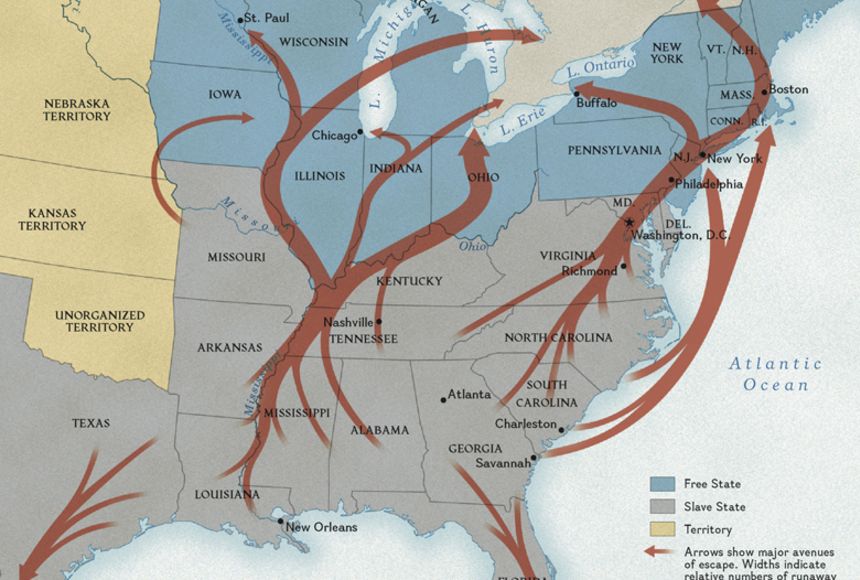This detailed map of a portion of the United States spans from Texas to the East Coast, reaching up to parts of Maine and down to the northern part of Florida. It is color-coded with three distinct colors denoting the status of each state: blue for Free States, gray for Slave States, and yellow for Territories. Important geographic markers such as the Atlantic Ocean and the Great Lakes (Michigan, Huron, Erie, and Ontario) are also visible.

A prominent legend in the bottom right corner specifies that blue represents Free States, gray represents Slave States, and yellow denotes Territories. It also contains a red arrow indicating "Arrows Show Major Avenues of Escape," with the width of these arrows representing the relative number of runaway slaves. The arrows predominantly originate from the gray Slave States, tracing various paths northwards to the blue Free States and Canada.

The map includes notable regions such as the Nebraska Territory, Kansas Territory, and Unorganized Territory to the west. It also features Free States like Iowa, Wisconsin, Illinois, Indiana, Ohio, Pennsylvania, New York, Vermont, New Hampshire, Massachusetts, and Connecticut. Slave States depicted include Texas, Louisiana, Missouri, Arkansas, Mississippi, Tennessee, Alabama, Georgia, South Carolina, North Carolina, and Virginia.

This map vividly portrays the historical routes taken by runaway slaves escaping to Free States and Canada, illustrating the significant human movement during this era. Various arrows indicate both the geographical paths and the intensity of these escapes, with thicker arrows marking routes with higher numbers of runaways, particularly routes passing through Ohio.